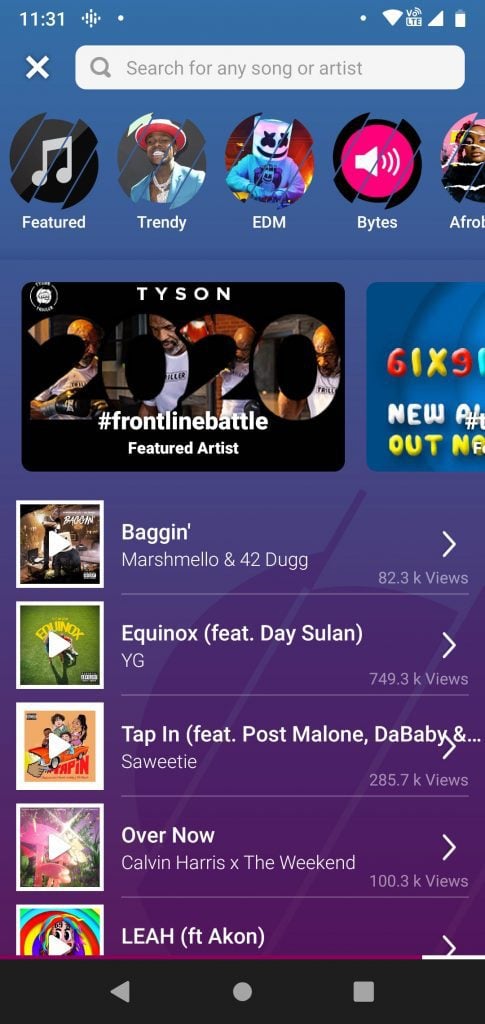The image depicts a music streaming interface with a variety of features. At the top, there's an ID number "1131" displayed prominently, alongside an "X" button for closing the interface and a search bar for user input. The interface showcases a trending EDM playlist, titled in all caps, and is highlighted by flashy bytes of graphics. Featured artist Tyson is promoting this playlist under the hashtag #FrontlineBattle.

The playlist consists of five songs curated for the listeners. The tracklist includes:

1. "Equinox" (featuring F.E.A.T. by Desalan) 
2. "Tap In" (featuring Post Malone, DaBaby, and others) 
3. "Over Now" 
4. "Leah" (featuring Akon) 
5. "F.T."

To the left of the list, there are thumbnail images of the album covers or artists, each with a triangular play button overlay, indicating the option to play the videos directly from the interface. The imagery is attributed to an artist named Baggin, contributing to the visual appeal of the playlist presentation.